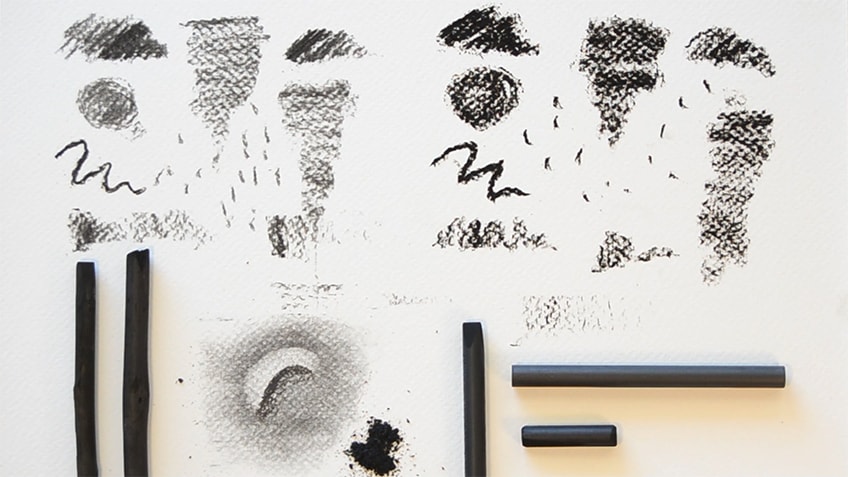The image captures an artist experimenting with black pastel and pencil crayons on a white sheet of paper. At the bottom of the image, there are five pencil crayons: two on the left that are nearly the same height, and three on the right, one of which is positioned vertically while the other two lie horizontally. The paper is filled with various shading tests where the artist has explored different levels of pressure and thickness. They have carefully placed dots and practiced smudging using their finger, suggesting they are experimenting with different techniques and ideas, possibly in preparation for a future artwork.